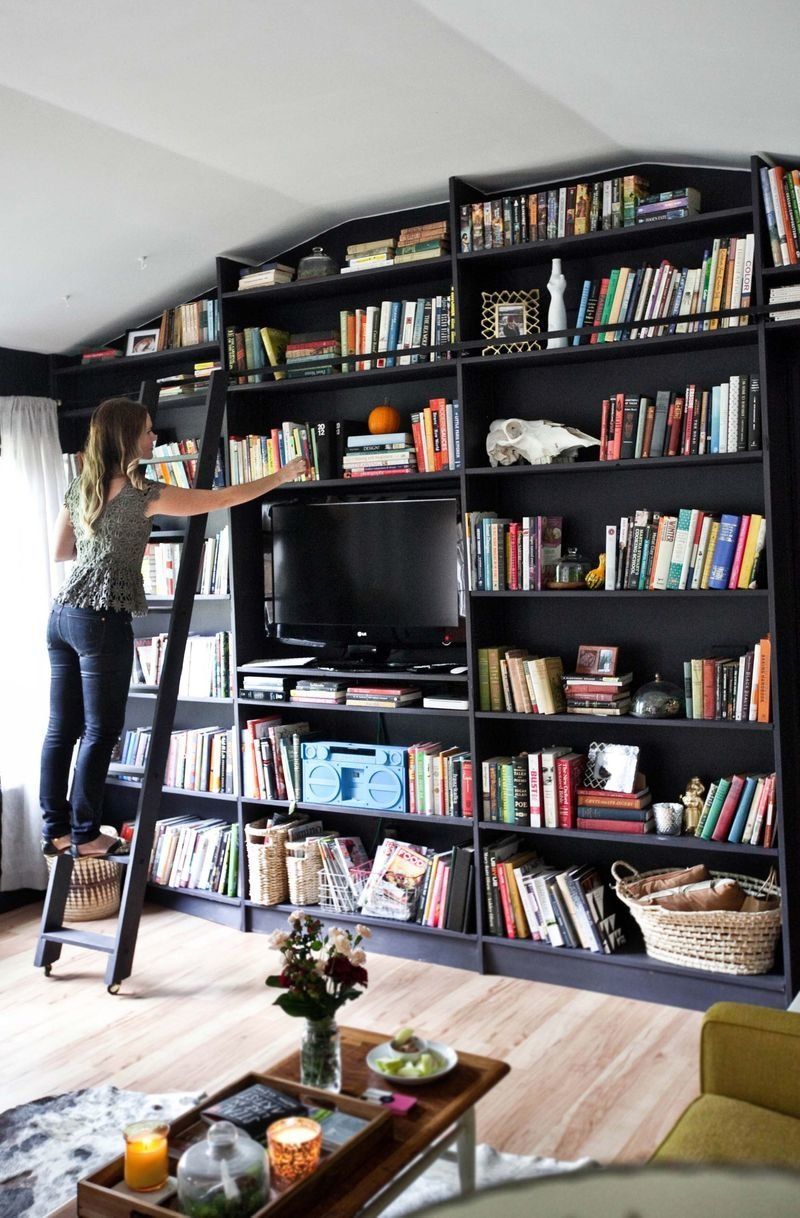The color photograph captures a well-lit living room with a very large black entertainment center that spans from the ground to the ceiling. This entertainment center features multiple shelves filled with a variety of items such as books, movies, a basket with pillows, picture frames, and a prominent skull. At the center of the entertainment unit is a flat-screen TV, approximately 40 inches in size, set within a square frame, with a blue radio positioned directly below it. To the left, a window with a white curtain allows natural light to flood the room. 

A woman stands on a ladder to the right, reaching for a book situated on a shelf above the television. She is dressed in a pale green blouse, blue jeans, and sandals, her long hair trailing down her back. The living room also includes a rectangular coffee table, adorned with white-pink flowers in a vase, a couple of candles, and a tray holding apple slices. Slightly visible in the bottom right corner is a pale yellow-orange couch, complemented by a white rug on the ground. The combination of these elements creates a warm and inviting atmosphere in the photograph.